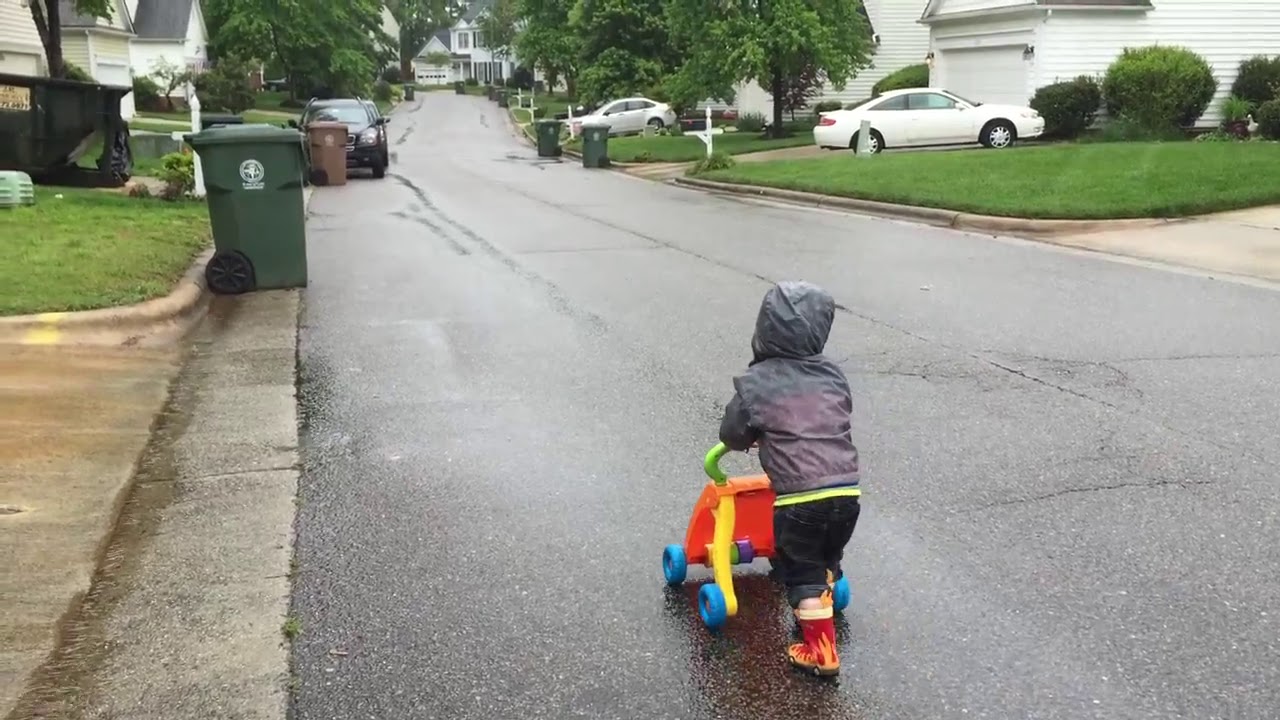In this photograph, we see a young child, likely around two years old, walking down a residential street on a rainy day. The child is at the bottom center of the image, pushing a brightly colored plastic stroller that is almost his height. The stroller features a lime green handle, a red back, an orange base, and yellow legs connecting to turquoise blue wheels both in the front and back. The child is wearing a gray windbreaker, blue denim pants, and vibrant red rain boots with yellow flames.

The neighborhood street is wet from recent rain, and the scene is filled with various objects and colors, including green and brown garbage pails, parked cars, and houses with driveways. Green trees and patches of grass are visible throughout. There are mailboxes near each house, adding to the quintessential suburban feel of the image.